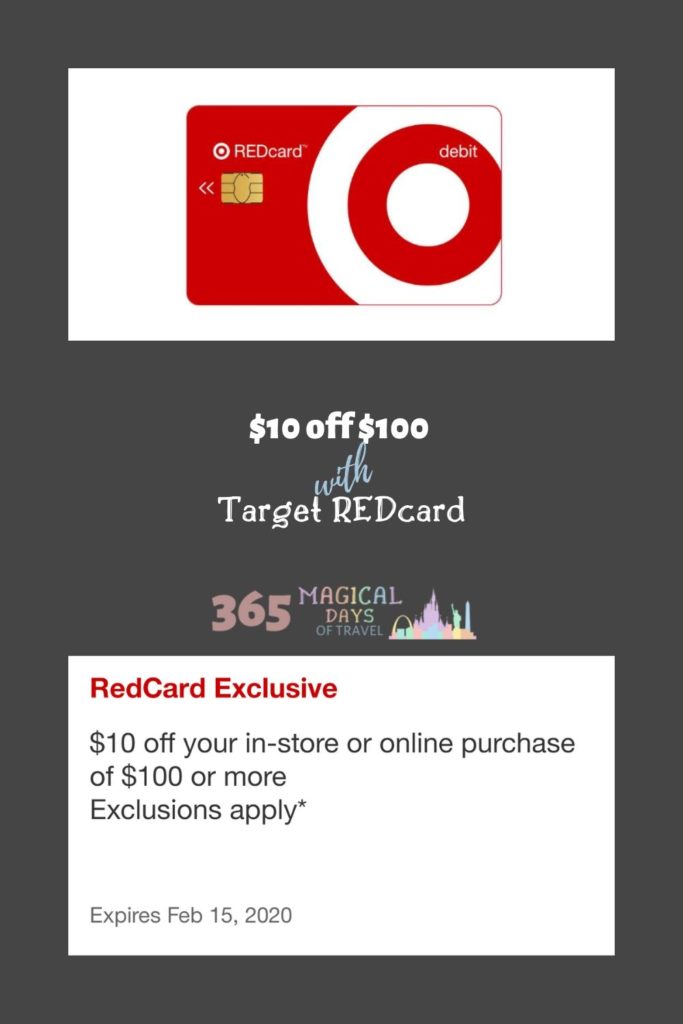The image has a black background with a white rectangle at the top. Within this rectangle is a prominently displayed Target REDcard, a red credit card featuring a white circle outline with a red and then white circle inside it. The card also includes a gold chip on the left-hand side. Below the card, text in white reads: "$10 off $100 with Target REDcard. 365 Magical Days of Travel." The backdrop behind this text includes a colorful, theme park-like design, adding a festive atmosphere.

Beneath this, there is another white rectangle of similar size and color. At the top of this rectangle, bold red text states: "REDcard Exclusive." Below this, in black text, it reads: "$10 off your in-store or online purchase of $100 or more. Exclusions apply.*" After a couple of line breaks, small text at the bottom notes the expiration date: "Expires February 15, 2020."